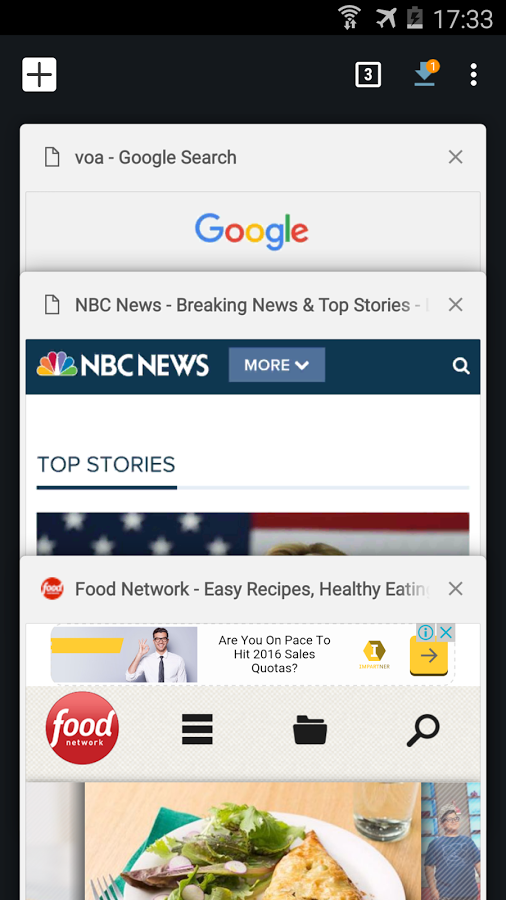The image displayed on the cell phone screen features a predominantly black background at the top, where a white square with a black plus sign is visible in the left corner. At the very top of the screen, the icons for Wi-Fi signal, airplane mode, and a nearly depleted battery are shown, along with the time, 17:33.

The screenshot also shows a white square with the number '3' inside it. Adjacent to this is a download icon accompanied by a circled number '1' and three small dots indicating additional options. The Google logo, featuring the classic multicolored lettering, is prominently displayed, with a page fold icon on its corner. Above "Google," it reads "VOA/Google search."

Below the search bar, there is a section labeled "NBC Breaking News and Top Stories," featuring the NBC logo with a peacock symbol in vibrant colors next to the text "NBC News." The "Top Stories" tab is highlighted in blue, underlined by a blue line. The background includes an American flag and part of a person's head.

Further down, an advertisement for the Food Network appears, promoting "Easy Recipes" and "Healthy Eating." Another ad below poses the question, "Are you in a pace to hit 2016 sales quotas?" At the bottom of the screen, a food-related section showcases a dish consisting of a salad and meat on a brown plate, topped with a clear glass cover. Accompanying the dish is a magnifying glass icon and a triple-line menu icon. Additionally, there is an image of a Caucasian man in a blue t-shirt, seemingly standing outside next to a building with numerous windows.